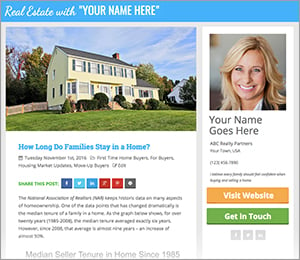In this detailed image, we see a computer screen displaying a real estate application. At the top, bold text reads "Real Estate," followed by the capitalized placeholder text "YOUR NAME HERE." Beneath this, there's an illustration of a yellow, two-story house adorned with five windows on its upper level, set against a backdrop of a clear blue sky. The image also prominently features the question, "How long do families stay in a home?" leading into an article discussing this topic.

On the left side of the screen, a row of social media icons — including Facebook, Twitter, LinkedIn, and Pinterest — allows users to share content across these platforms. Each icon is neatly arranged in squares, enabling easy selection for posting.

To the right of the main content, there's a sidebar featuring a profile section. This includes a profile picture of a professional-looking blonde woman, likely in her 30s, alongside her name, written as "YOUR NAME HERE." Below her name are two interactive buttons: "View Website" in brown and "Get in Touch" in green, providing options for further engagement. The social media logos within this section are subtly shaded, maintaining a cohesive and visually appealing design.